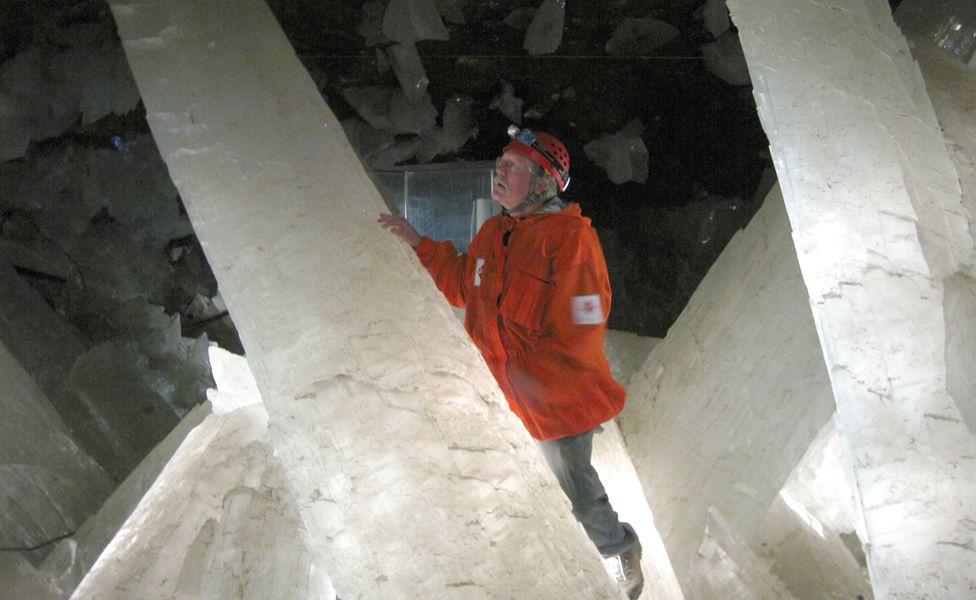In this photograph, an older white man with gray hair, a gray mustache, and glasses is standing inside a cave adorned with massive, naturally formed quartz crystals. He wears a red helmet with a headlamp, a deep orange jacket, gray pants, and hiking shoes. The man gently rests his right hand on one of the monumental crystal columns, which are about four times his size and lean slightly to the left. The crystals, standing prominently in the foreground, catch and reflect light, illuminating the immediate area around him. Beyond him, the cave recedes into darkness, punctuated by more crystal formations emerging from the walls and floor. The scene suggests a location of awe-inspiring natural beauty, possibly in a cave in Mexico, which is now off-limits to visitors. The overall image, though not of high resolution, captures the man's quiet contemplation of these immense and luminous mineral formations.